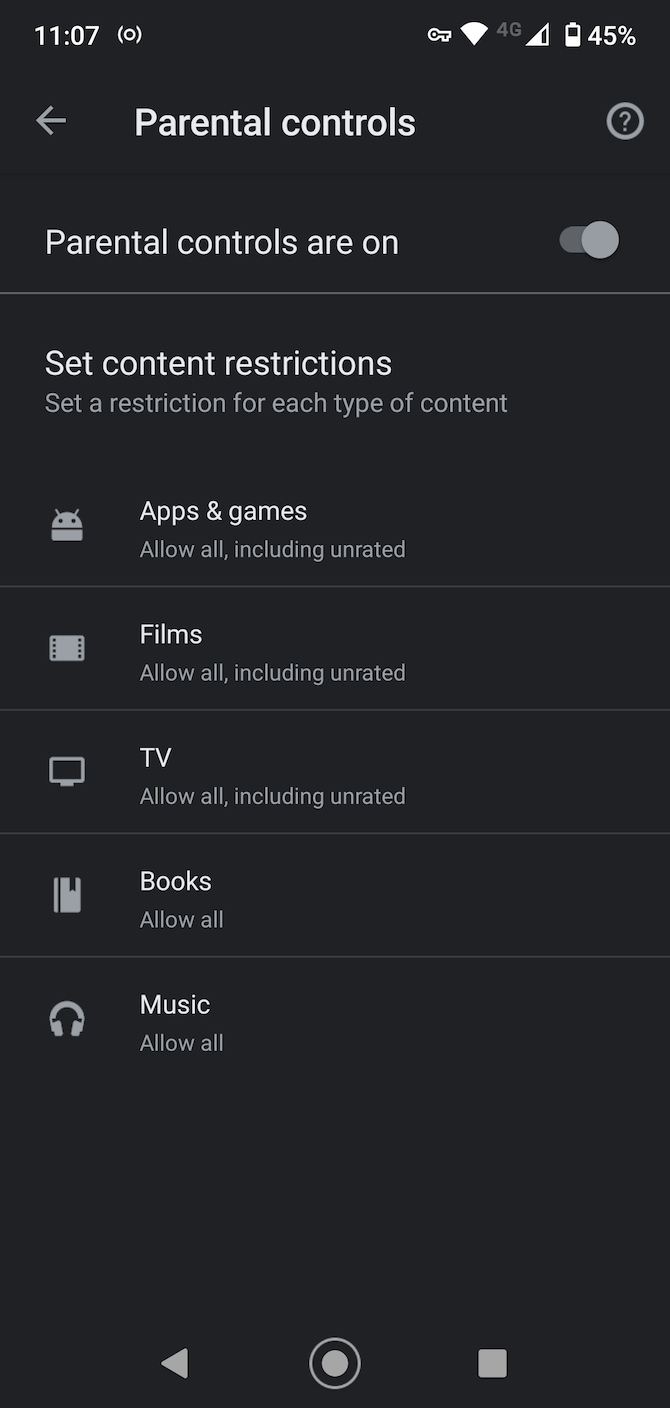The image displays a detailed parental control settings screen on a device. At the top of the screen, the list starts with "1107" followed by icons indicating key features: Wi-Fi, 4G, and battery status at 45%. Parental controls are activated, as indicated by a question mark next to the label.

Under parental controls, there are options to set restrictions for various types of content, accompanied by icons and descriptions:

- **Apps and Games:** "Allow all including unrated." An Android icon is shown beside this option.
- **Films:** An image of a film strip with the label "Allow all including unrated."
- **TV:** TV icon with the setting "Allow all including unrated."
- **Books:** A book icon with the setting "Allow all."
- **Music:** A music note icon with "Allow all."

Additionally, the interface includes navigation elements such as a left arrow, circle, and center icons. The background appears to be very grayed out, almost dull, with a noticeable pink safety icon. 

Overall, the screen provides a comprehensive control mechanism for various types of media content, allowing users to manage what can be accessed on the device.